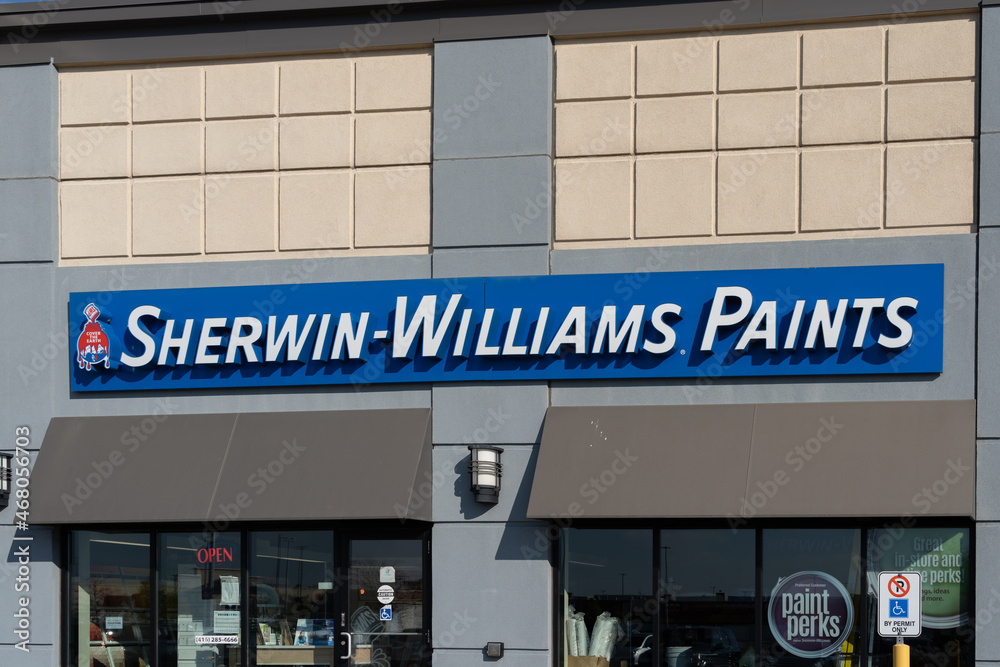This detailed illustration depicts a highly realistic storefront of a Sherwin-Williams paint store. Dominating the upper section of the image, the storefront facade is characterized by large, gray concrete tiles centrally positioned, flanked by very light beige sections on either side. Prominently displayed across the width of the shopfront is the expansive Sherwin-Williams sign, featuring a bold blue background with the brand name spelled out in large white letters, accentuated by a subtle dark shadow to enhance visibility.

To the left of the sign rests the iconic Sherwin-Williams logo: a globe enveloped by red paint dripping over it. Below the sign, the storefront is outfitted with shutters over its windows. There are two windows visible — one on the left and one on the right. The right window is partially adorned with a promo decal reading "Paint Perks." Adjacent to this right window, a parking area is indicated by a signage system. One sign is a white rectangle with a red P crossed out, signifying no parking, next to another sign denoting a blue square with a schematic drawing of a wheelchair, indicating a handicap parking spot.

In the lower-left corner of the image, the text "Adobe Stock" subtly alludes to the source of the illustration, confirming it as a stock image.